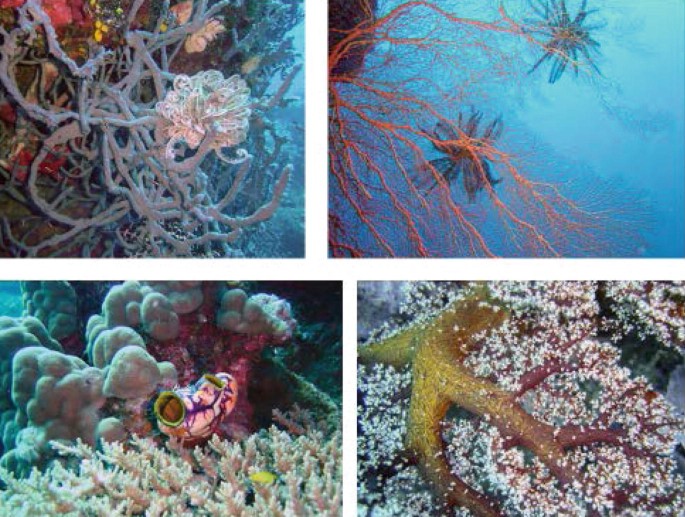This image grid showcases four distinct underwater photographs arranged in a two-by-two layout, each capturing a unique aspect of underwater sea life. 

The top left photograph displays an intricate tangle of gray coral, resembling branches or tentacles with speckles of white, yellow, and red amidst a backdrop of blue ocean water. The top right photograph features spindly, delicate, and root-like orange and pink corals extending into the water, evoking the appearance of the veins within a human lung. Here, two sea stars, akin to spiky, leaf-like forms, float nearby.

In the bottom left photograph, fluffy, cotton ball-like white corals dominate the scene, accompanied by other coral formations of varied textures and colors. A mysterious sea creature or additional coral type is discernible in the center. Meanwhile, the bottom right photograph captures a starfish, golden in hue, lounging atop a bed of white, flowery coral interspersed with red, vein-like extensions and barnacle-like growths.

Together, these images paint a vibrant and detailed portrait of underwater coral reefs, highlighting the diverse and intricate forms of marine life within this aquatic environment.